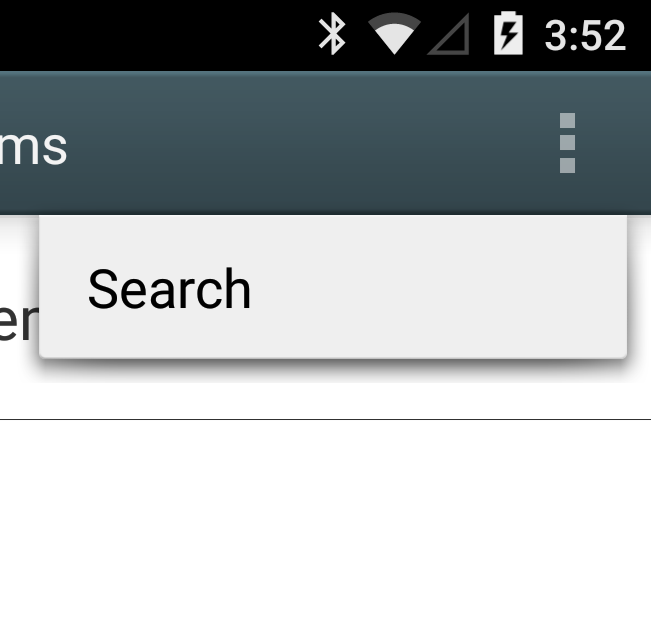The screenshot appears to be from a mobile phone or tablet interface. In the top-right corner, there are several white icons prominently displayed on a status bar against a black rectangle background. These include a strong Bluetooth signal meter indicating approximately an 85% connection strength, a downward-pointing triangle to the right, and a battery symbol featuring a lightning bolt, showing the battery percentage at 3:52 PM.

Below this status bar, a dark greenish-gray rectangle contains three ellipses and the partially visible text "MS." Underneath, another grayish rectangle displays the word "Search" in black text on a lighter gray background. Behind this, white space with partially visible letters, potentially "ER" or "EM," is observed, suggesting it could be part of a word or heading. This is followed by a long black line at the bottom of the screen, which signifies a search bar.

This detailed interface likely belongs to an application or setting screen, given the layout and content presented.